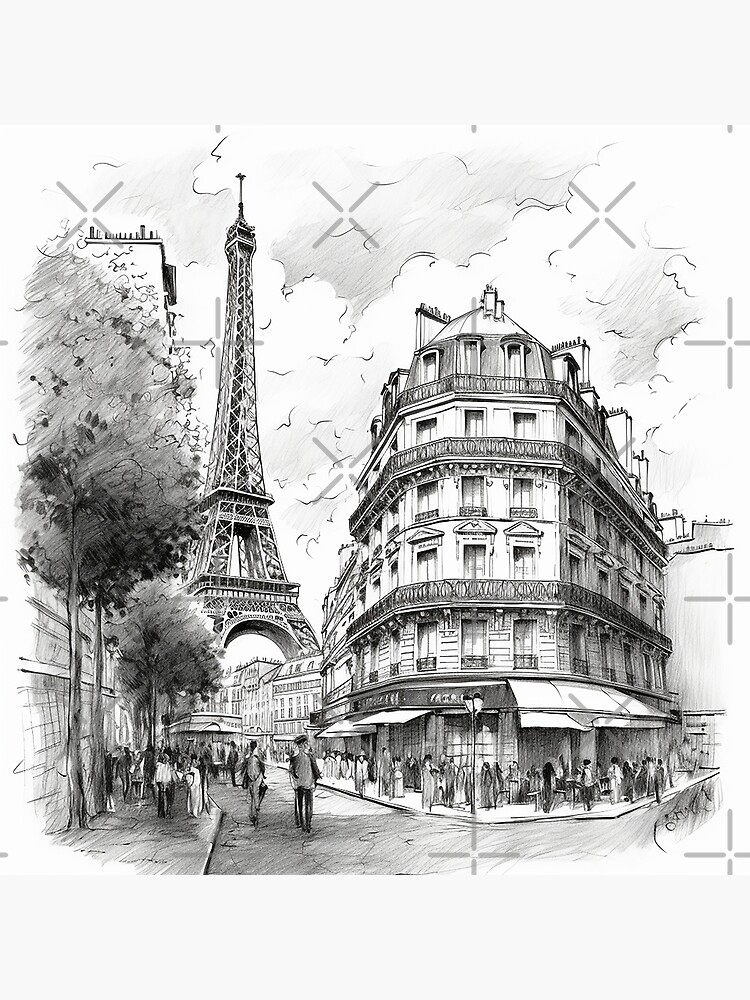The image is a detailed black and white hand-drawn sketch of a Parisian scene centered around the Eiffel Tower. The scene includes various artistic elements such as watercolor accents, pencil, and charcoal, which lend it a shadowy and textured appearance. The Eiffel Tower stands tall in the background, rising above a bustling cityscape.

In the foreground and mid-ground, larger buildings surround the Eiffel Tower. Prominently, a grand six or seven-story corner building with large balconies curving around its facade dominates the scene. This building flanks both sides of the street, creating a cafe-like ambiance as numerous silhouettes of people, drawn in simple black and white, traverse the sidewalks and streets. Their faces lack detail, emphasizing the sketch’s stylistic focus on movement and atmosphere rather than individual features.

To the left, three trees line a busy street filled with pedestrians, while additional buildings extend toward the base of the Eiffel Tower. The top center of the sketch is graced by clouds, adding depth to the sky. Subtle signatures of the artist, "David Burstein," appear twice—one embedded in the clouded background stretching from the Eiffel Tower to a neighboring building, and another in the lower-right section, likely marking the authenticity of the artwork.

Overall, the sketch beautifully captures the lively and timeless essence of Paris, blending iconic architecture with everyday urban bustle.